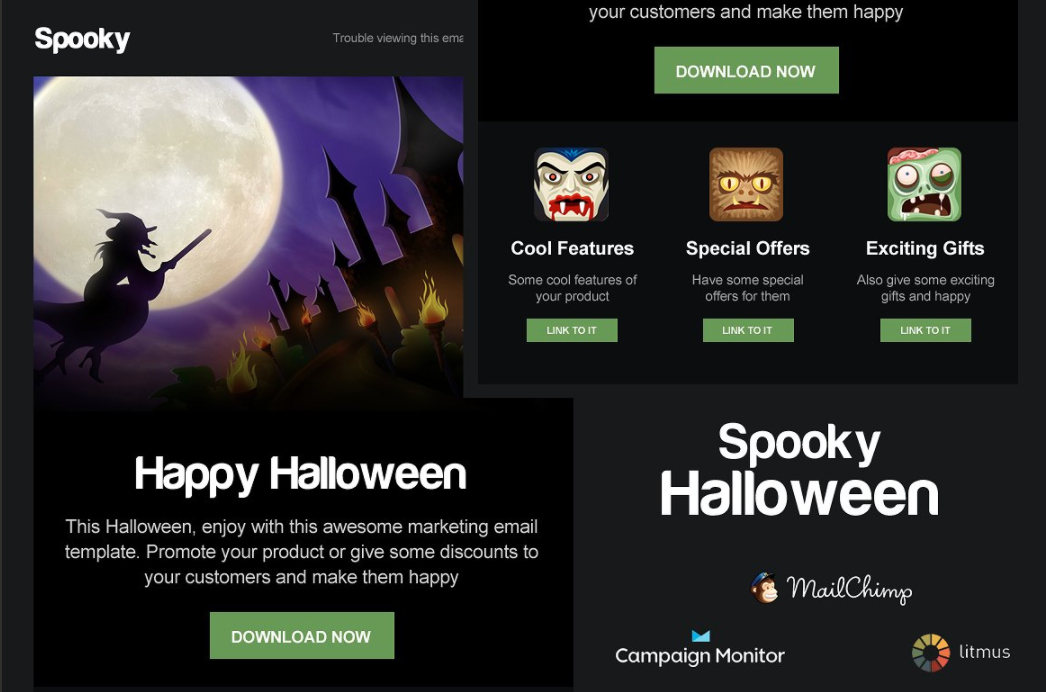Photographic Image Description:

The image captures a vibrant web page themed around Halloween, designed to promote a marketing email template. 

In the upper left-hand corner, the word "spooky" is prominently displayed in white font. To the right, a pop-up box appears with the message: "Your customers and make them happy," accompanied by a green "Download Now" button.

The central part of the web page showcases three cartoon characters, each representing different promotional features:

1. **Dracula**: Characterized by blue hair shaped into a distinctive widow's peak, Dracula has red eyes, fangs, and blood dripping from his mouth. He introduces the section titled "Cool Features," which highlights some appealing aspects of the marketed product, including a link to learn more.

2. **Werewolf**: Representing "Special Offers," this character suggests exclusive deals available to customers, complete with a link for more details.

3. **Monster**: Symbolizing "Exciting Gifts," this character encourages offering exciting gifts to customers to make them happy, with an associated link.

The lower section of the webpage features a dramatic graphic of a witch flying on a broomstick in front of a full moon, heading towards a castle illuminated by fiery torches. The sky is depicted in deep shades of blue and purple. Below this scene, text in a playful font reads: "Happy Halloween," followed by a message encouraging users to enjoy Halloween with the "awesome marketing email template" to promote products or offer discounts. Another green "Download Now" button lies beneath this festive invitation.